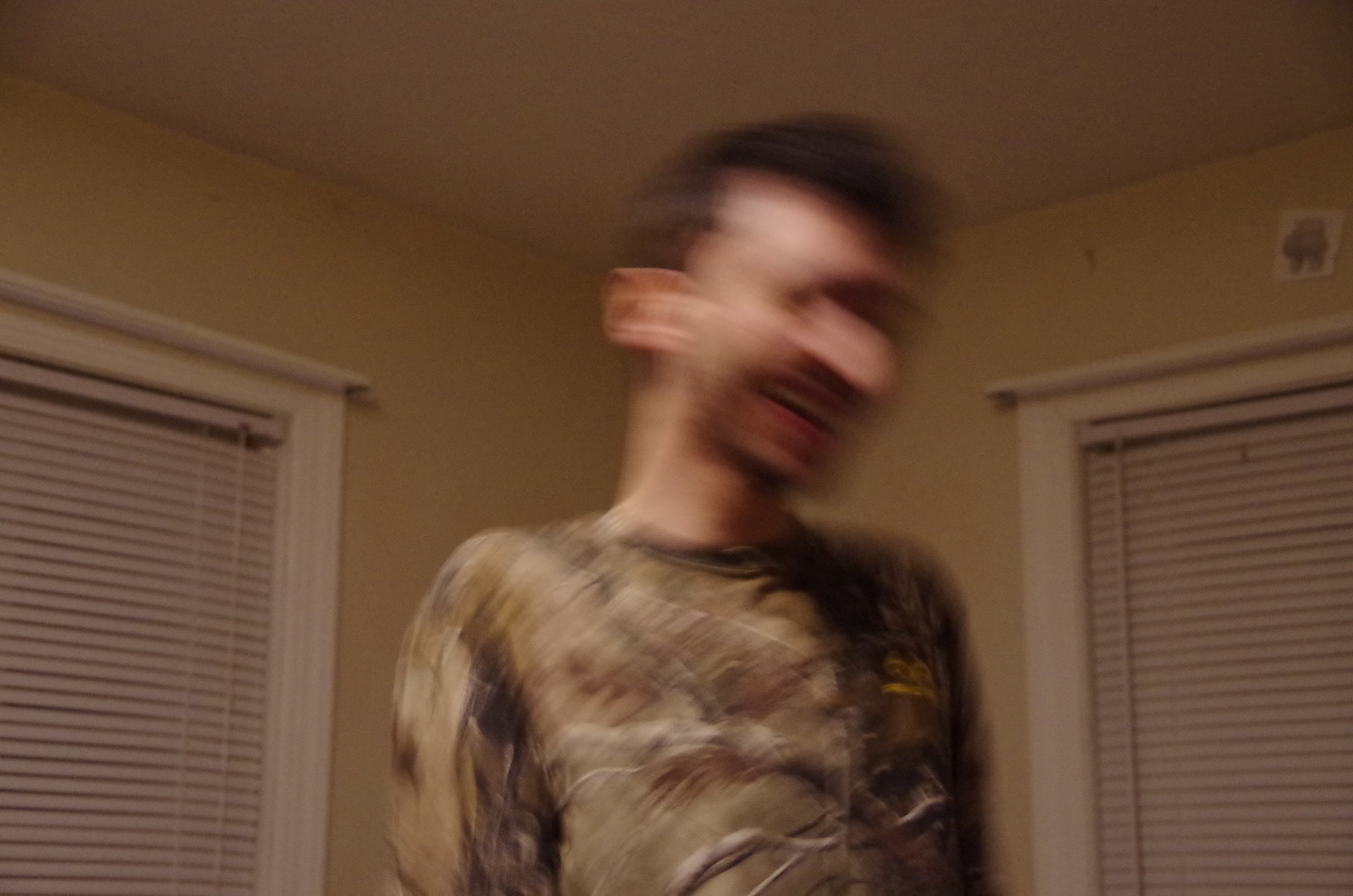The photograph captures an incredibly blurry image of a slender man standing in a room. His head appears to be moving rapidly, giving the illusion of multiple ears and a distorted face, with indistinct features such as short brown hair and a hint of facial hair, possibly a mustache and beard. His mouth is open, revealing the top row of his teeth, suggesting he might be laughing. He is dressed in a long-sleeved, woodland camouflage shirt, characterized by a mix of brown and beige colors, and a blurred yellow logo. The background reveals a room with beige or pale yellow walls, and two windows equipped with white-framed horizontal blinds. The windows’ trim and the ceiling are also white, contributing to the room's neutral color palette.